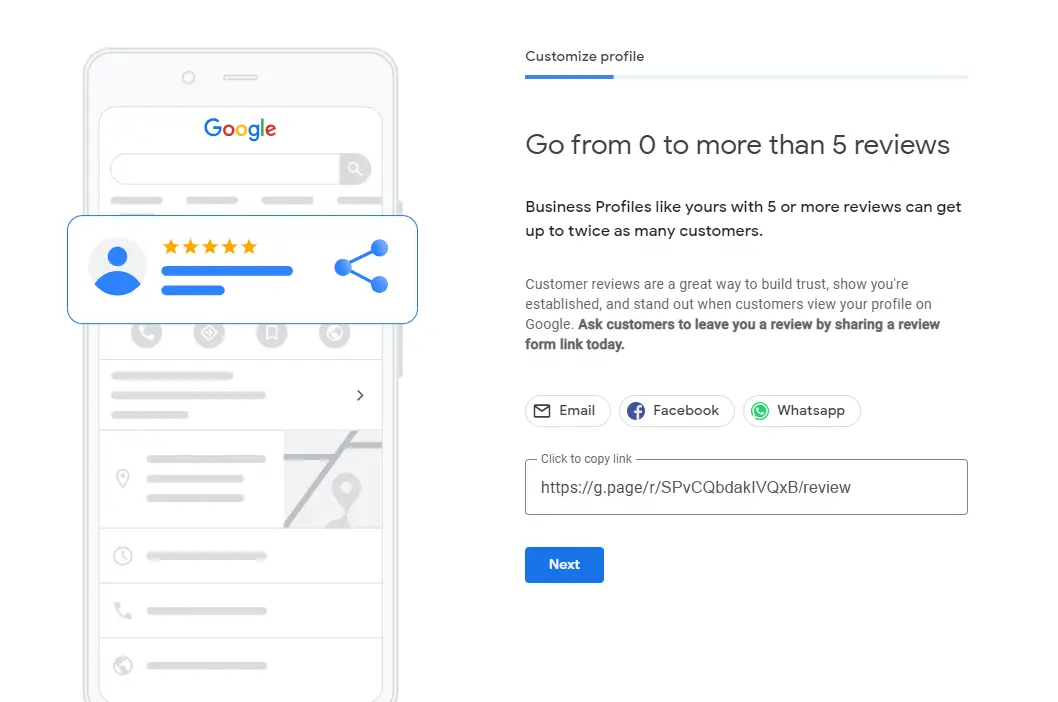The image is a slightly horizontally rectangular frame showcasing the outline of a cell phone interface on the left side. At the top center of the displayed mobile screen, the Google logo is prominently featured. Moving to the right side of the frame, a custom profile section is visible at the top. Below this section, a message highlights the importance of customer reviews, mentioning that business profiles with five or more reviews can attract up to twice as many customers. The text explains that customer reviews are essential for building trust, establishing credibility, and standing out to potential customers viewing your profile on Google. 

In bold letters, the image encourages businesses to ask customers for reviews by sharing a review form link. Underneath this call-to-action, there are three buttons arranged side-by-side, labeled "Email," "Facebook," and "WhatsApp," designed for sharing the review link through these platforms. Below these buttons is a field with the text "Click to copy link," followed by a URL: https://g.page/.R.S.P.V.C.Q.BDAKL.V.Q.X.B.R. At the bottom of the frame, a blue "Next" button is displayed.